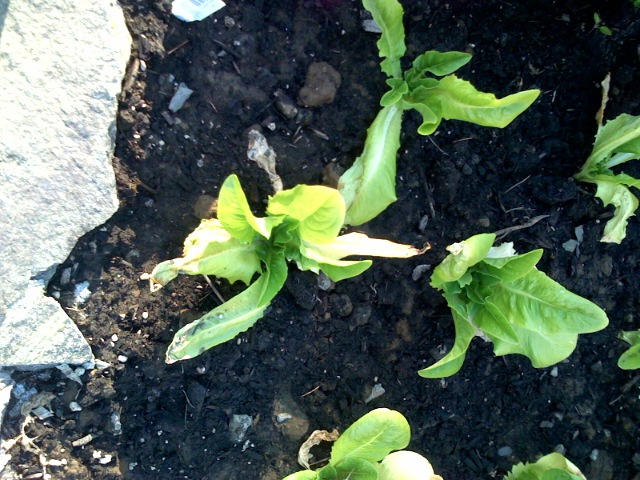This overhead daylight photograph captures a small vegetable garden bed encircled by jagged gray and tan stones, potentially flagstones or limestones. The garden bed features freshly turned, rocky, dark brown soil with various clumps and some lighter patches. Small bright green lettuce plants, just sprouting with four or five tender leaves, are scattered in somewhat regular rows across the soil. Sunlight bathes the scene from the left side, casting natural light over the garden and highlighting the textural contrasts between the dark soil, the bright green sprouts, and the gray stones. The plants appear delicate and new, with some smaller sprouts just beginning to emerge, indicating a freshly cultivated garden space.